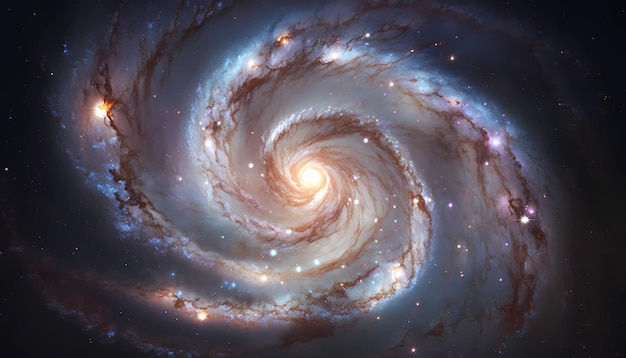The image portrays a stylized representation of a spiral galaxy, predominantly depicted using a mix of white, brown, and pink clouds interspersed with bright, multi-colored lights symbolizing stars or solar systems. Radiating outwards from a prominent, luminous yellow circle at the center are four spiral arms, depicted in hues of blue and reddish tones. Stars of various colors—pink, blue, yellow, and white—are scattered throughout these arms, adding vibrant points of light against the dark backdrop. The background edges of the image, specifically at the four corners, are primarily black, dotted with small white stars, enhancing the depth and the cosmic setting. The center of the galaxy, where everything seems to rotate around the yellow core, is the brightest part of the image. There appears to be an additional bright mass, possibly another galaxy, situated on the left side, which adds to the richness of the celestial scene. This detailed and mesmerizing image, which might be a painting or a graphically created picture, captures the grandeur and complexity of cosmic structures.